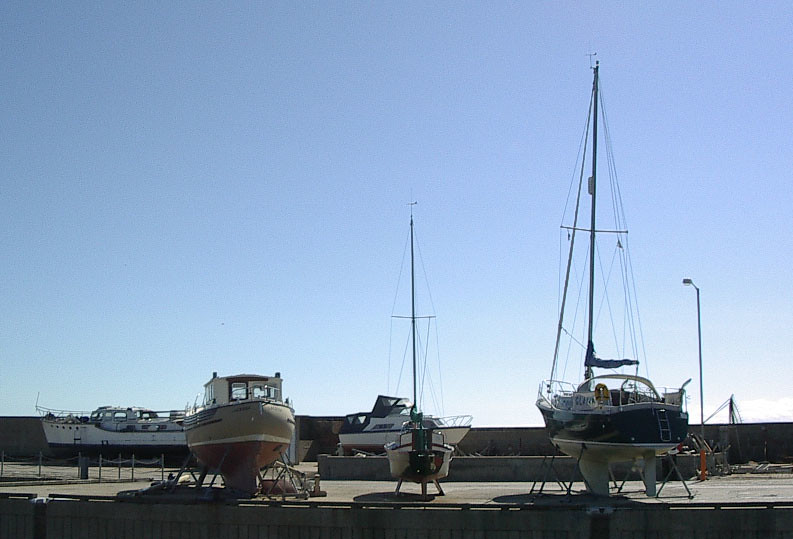This image captures four boats resting on stands in a dry dock, situated on a concrete slab. The boats are all out of the water, making their keels clearly visible. The vessel on the far right is a medium-sized sailboat, easily identifiable by its mast, rigging, and furled sail. Adjacent to it is another sailboat, but this one is smaller. Next to the smaller sailboat is a motorboat, featuring a cabin with windows—it appears to be an older wooden model. Beyond these, in the background, another sailboat can be spotted by its mast, and a motorboat, likely a fishing boat or possibly a yacht, stands further back with a prominent cabin on top. The sky overhead has a light, steel-blue hue, and a street light is visible in the right-hand corner of the dry dock. This setting suggests a tranquil marina or boatyard scene, where personal watercrafts are being stored or maintained.